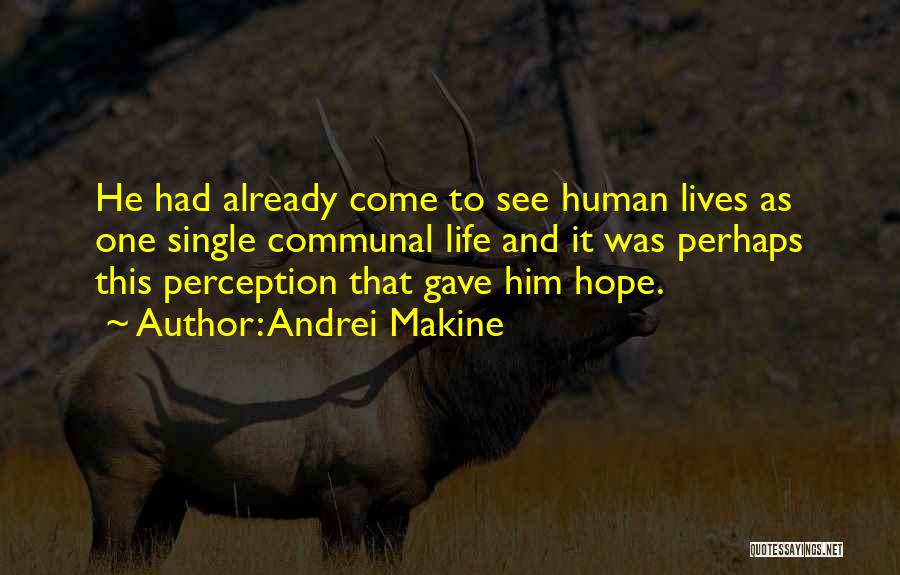In the center of the image is a quote written in yellow text: "He had already come to see human lives as one single communal life, and it was perhaps this perception that gave him hope." The quote is attributed to Andre Makine and additionally includes the names "Her Colon and Ray McKee." The background features a somewhat darkened photo of a swamp deer standing in yellowish-orange grass fields, with a tree visible. Towards the bottom right corner, there is a graphic on a white background with the website name "quotesayings.net."